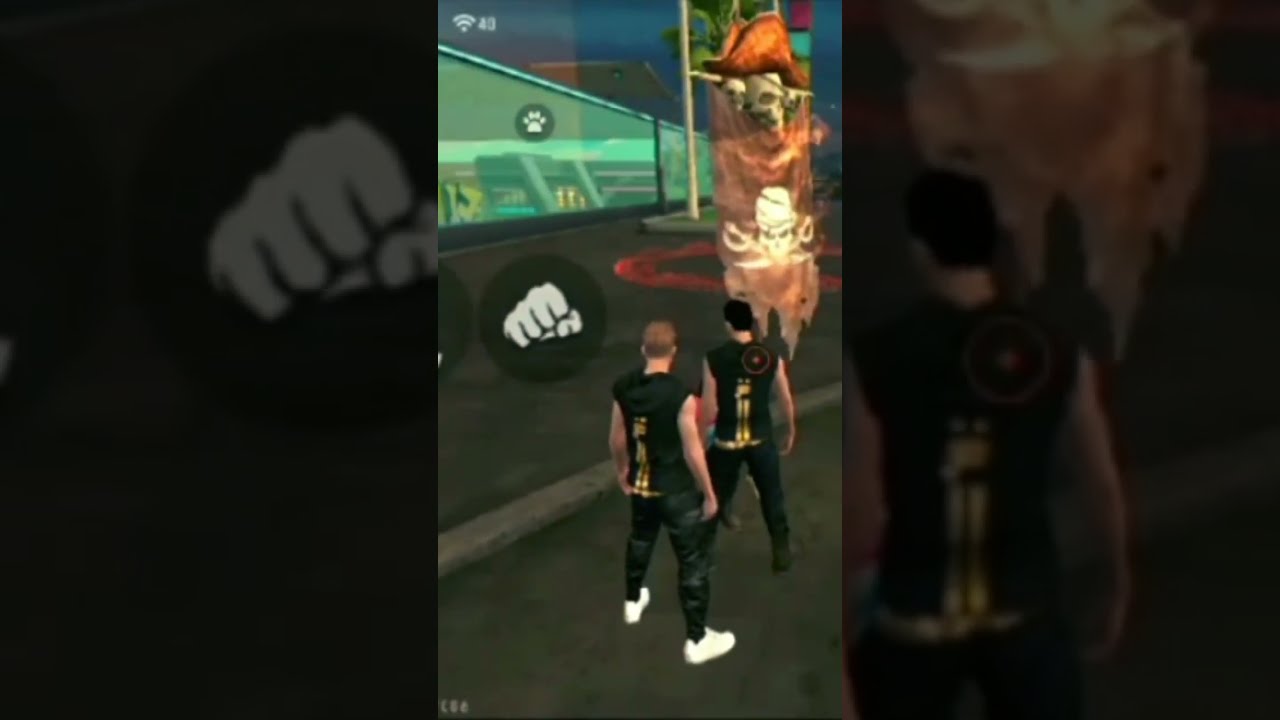In this detailed image, we have a screenshot from a 3D video game, likely designed for mobile devices, as indicated by the Wi-Fi logo in the upper left corner. The scene features two male characters standing confidently on a curbside street, their backs facing the viewer. Both characters are dressed identically in green sleeveless hoodies adorned with a gold design on the back and matching green pants. The closer character has light brown hair and is wearing white sneakers, while the further character has black hair and dark sneakers. 

They stand in front of a prominent pirate-themed emblem featuring a skull and crossbones motif on a banner, which is illuminated and vividly colored in red, orange, yellow, and white. The background reveals a black glass-like environment with a sky fading into twilight hues. Additionally, game interface elements are visible, including a circle with a fist icon and another smaller circle with a paw print. This immersive setting suggests an adventurous, possibly combat-oriented game.